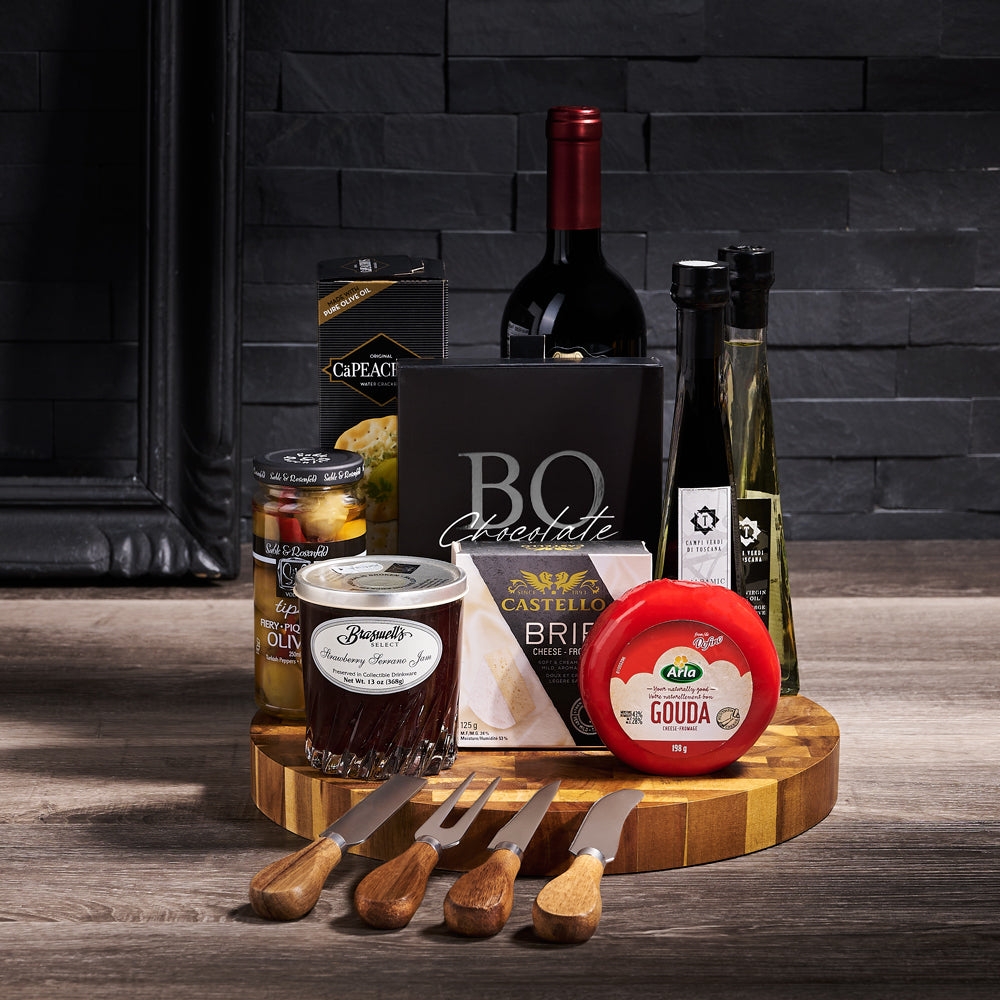This detailed close-up product photograph showcases a meticulously arranged cheese and charcuterie board set against a visually striking black-painted brick wall and complementing whitewashed wooden floor. The items are artistically displayed on a thick, round wooden cutting board. The setup includes four wooden-handled serving utensils— a knife, a pointier knife, a two-tined fork, and a flat bladed tool—leaned strategically on the board. Adjacent to this, a black-painted wooden mirror leans against the brick wall, partially visible on the left. 

The board hosts an impressive selection: a glass jar of strawberry serrano jam with a silver lid, a bright red wax-coated wheel of Arla Gouda cheese, a box of Castello Brie, a glass jar of olives with a black cap, and a large black box labeled Bow Chocolate. There’s also a bottle of wine with a red wrapping around the top, only the neck visible from behind the Bow Chocolate box. To the right, another black box presumed to be crackers adds visual depth, while a jar of vinegar and a bottle of olive oil, both with black caps, complete the ensemble. The overall presentation is both elegant and inviting, perfect for any sophisticated gathering.